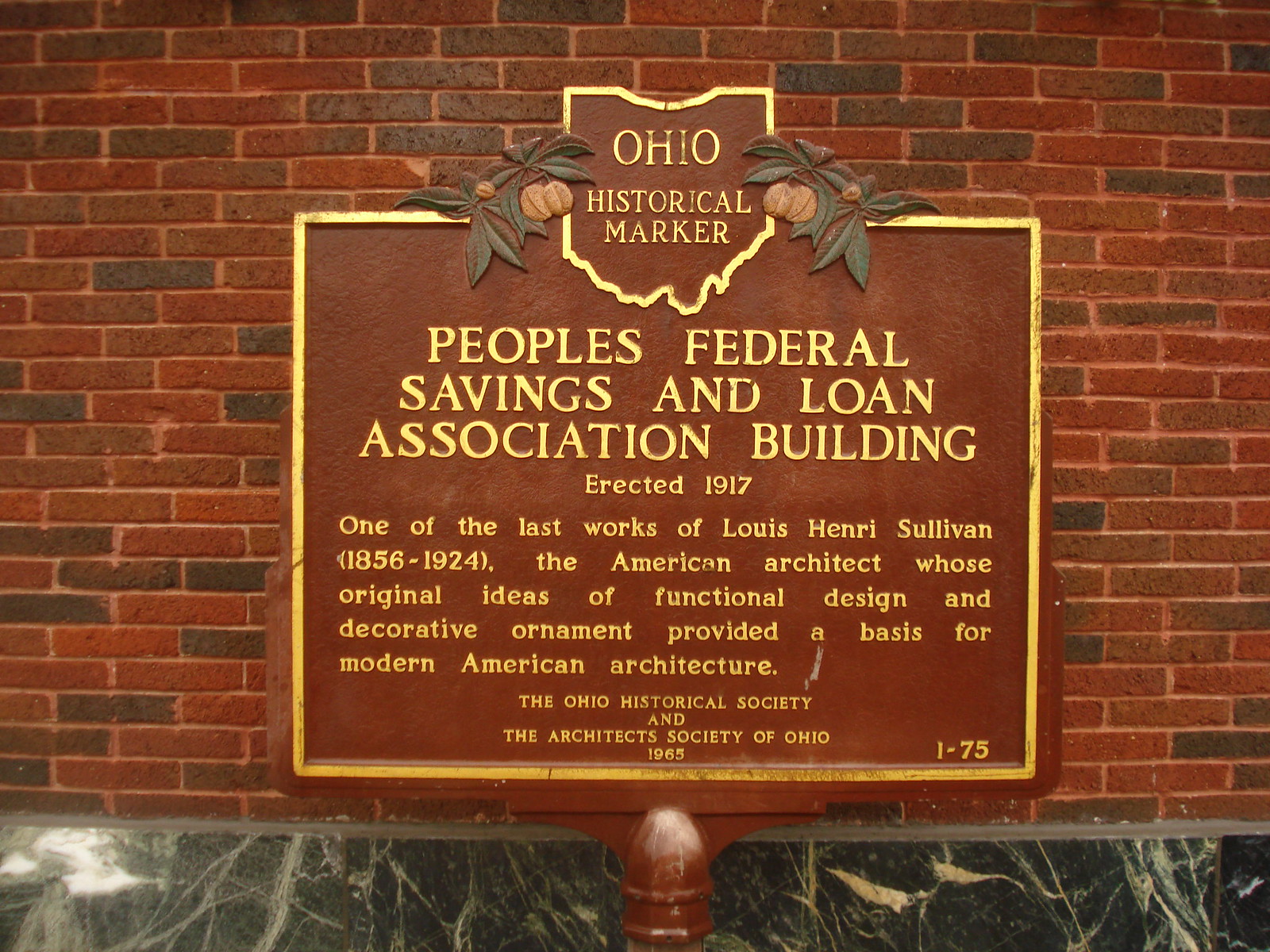The image depicts a notable red brick building, accented with brownish-red hues and green granite at its base. Prominently in front of the building is a red metal sign mounted on a red pole, featuring the yellow-bordered shape of the state of Ohio at the top, along with decorative leaves and fruit. The sign declares "Ohio Historical Marker" and prominently states "People's Federal Savings and Loan Association Building," erected in 1917, as one of the best works of esteemed American architect Louis Henry Sullivan (1856-1924). Sullivan's innovative designs in functional construction and ornamental detailing significantly influenced modern American architecture. Additionally, the bottom right corner of the sign includes the designation "I-75" and credits the Ohio Historical Society and the Architects Society of Ohio, 1965. On the ground, flanking the sign, are two small flowers, adding a touch of natural beauty to the scene.